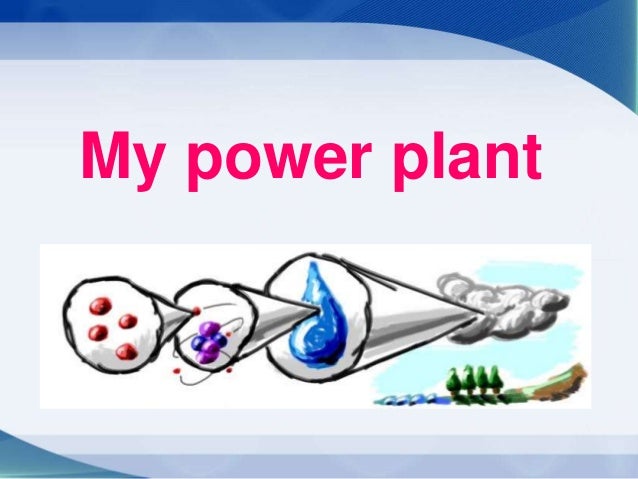The slide, likely part of a PowerPoint presentation, titled "My Power Plant" in pink text at the top center, is framed by blue accents, featuring a border with a curved blue gradient that is thicker on the right and a small blue triangle in the bottom left. The background is mostly white with light blue strips at the top and bottom. Below the title, the image consists of a series of conical structures that appear to magnify elements from right to left. The rightmost structure depicts a large water droplet beneath a white cloud, with a diagram showing trees, a body of water, and a brown mountain below. The middle conical structure contains an atom with its nucleus and electrons, rendered in purple and blue, while the leftmost structure features several red dots, resembling particles or electrons. The overall aesthetic is digital, styled to look like a child's crayon drawing, and appears to illustrate the process of how water droplets in clouds might be broken down to harness power, making it suitable for a school assignment on power plants.